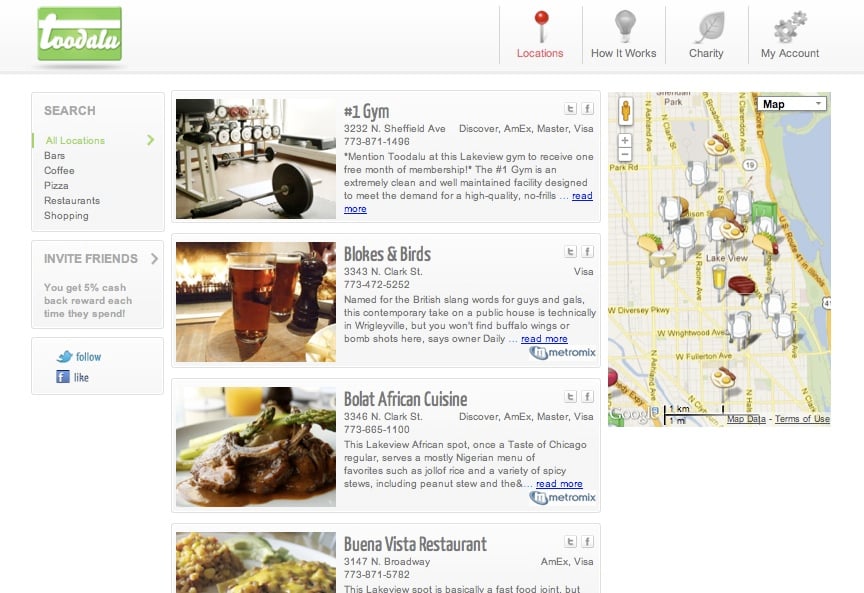Screenshot of a web page from a platform called "Tu Dalu," characterized by its green background and white cursive logo resembling a gift box. At the top of the page are navigation options including "Locations," "How It Works," "Charity," and "My Account." There's also a search bar with categories such as "All Locations," "Bars," "Coffee," "Pizza," "Restaurants," and "Shopping." Users can invite friends and earn a 55% cashback reward each time friends spend, as well as follow or like the page.

The page prominently features a map highlighting various cities, including Lakeview. It appears to be set in Chicago. The first recommendation is "Number One Gym" located at 3232 North Sheffield Avenue. By mentioning "Tu Dalu" at the gym, users can receive one free month of membership. The gym is described as an extremely clean and well-maintained facility meeting high standards of quality.

Next is "Blokes and Birds," a contemporary pub located in Wrigleyville, Chicago, named after British slang for "guys and gals." Unlike typical pubs, this establishment doesn't serve buffalo wings or bomb shots, as noted by the owner.

Another recommendation is "Olad African Cuisine," a Lakeview spot that offers a menu primarily featuring Nigerian dishes, such as Jollof rice and a variety of spicy stews, including peanut stew.

Finally, there's a mention of "Vino Vista Restaurant," presumably another noteworthy dining option in the area.

This detailed and well-structured layout provides users with insightful information about local businesses and rewards offered through the Tu Dalu platform.